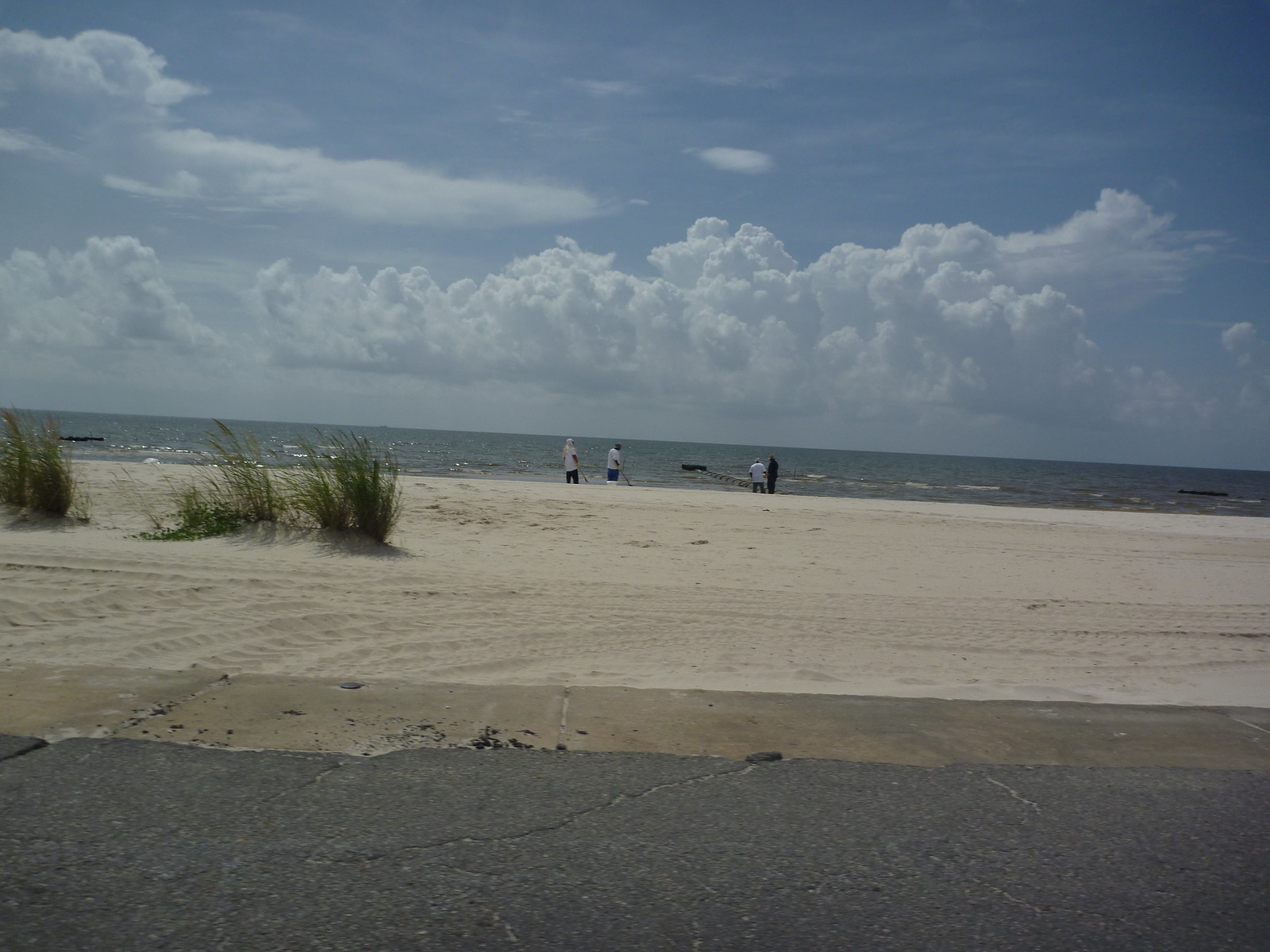This rectangular photograph captures an exterior beach scene from the perspective of a nearby cement road. In the foreground, the cracked black asphalt transitions into light brown sand almost immediately, accompanied by a narrow strip of tan sidewalk. On the left side of the image, clumps of tall, green dune grass sway gently in the wind.

Further back, the tranquil shoreline meets a dark blue sea, with gentle waves creating a sense of subtle activity in the water. Dominating the background, the sky is a bright blue adorned with scattered, fluffy white clouds.

At the edge of the beach, four individuals are positioned near a small pier. Three of them are dressed in white tops, while the fourth is clad in dark clothing. One person wears a white hat. These figures are possibly engaged in fishing or metal detecting, although their specific activities remain difficult to determine from the photograph’s distance. They stand facing the sea, seemingly absorbed in the serene coastal landscape.